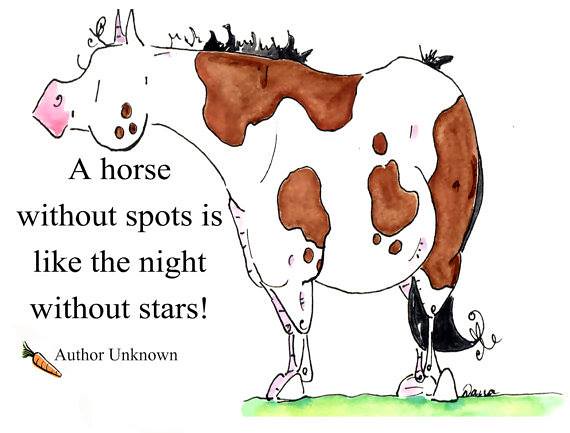In this charming watercolor illustration, a white cartoon horse with brown spots stands on a patch of green grass. The horse, facing left, has a pink muzzle and a mane and tail that are primarily black, though somewhat crudely drawn, adding to its whimsical appeal. Beside the horse, in black letters, the caption reads, "A horse without spots is like the night without stars!" Underneath this quote, an orange carrot with a green top is depicted, accompanied by the phrase "Author Unknown." The grass beneath the horse features an illegible signature, suggesting a personal touch to this delightful drawing.